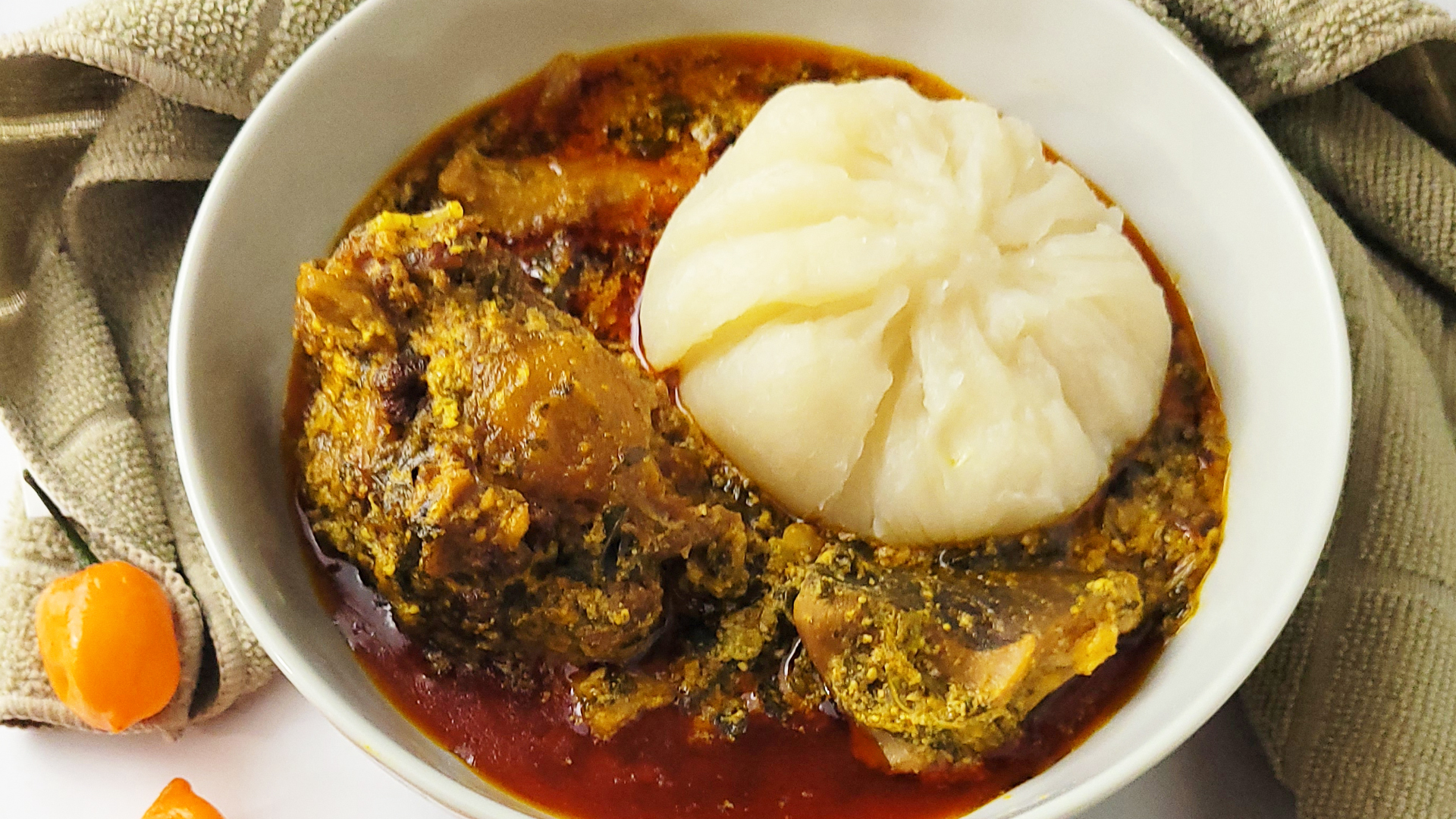This image shows a white bowl, potentially made of porcelain or plastic, resting on a white countertop and partially surrounded by a light, tan towel. The bowl contains a dessert-like dish featuring a vivid red liquid at the bottom, a mysterious brownish tan blob that could be meat or something coated in cinnamon, and a prominent white dollop of an unknown substance, which might be mashed potatoes, ice cream, or cream cheese, characterized by pressed lines. Two yellowish, grape-sized fruits or vegetables with small stems appear to the bottom left of the bowl, adding to the enigmatic nature of the contents.